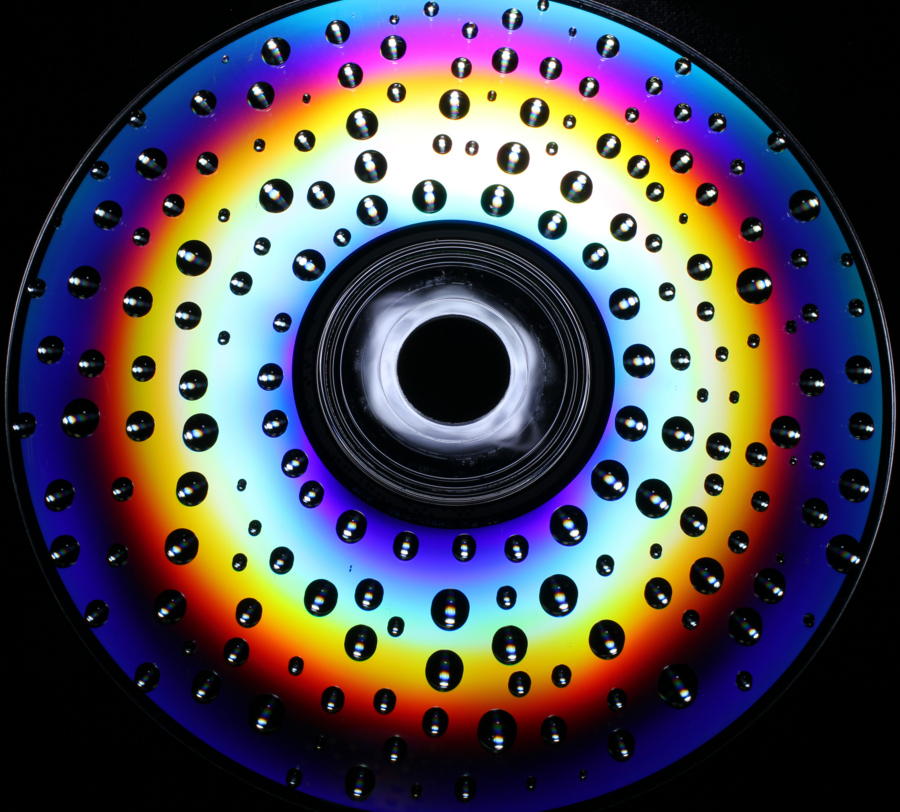This vivid photograph features a large, detailed circle against a black background, exuding a spectrum of vibrant colors arranged in an ombre pattern. The colors transition seamlessly from green to blue, red, yellow, aqua, purple, and various shades in between, forming concentric rings. At the center of the circle lies a black core surrounded by a white, almost ghostly ring, reminiscent of an iris and pupil. Encircling this central point are numerous small black dots or spheres, many with shiny elements, giving the appearance of droplets or bubbles. These elements contribute to a striking, almost eye-like design. The outer edges of the circle are bordered by darker hues, lending a sense of depth to the image. The entire composition is devoid of text or human figures, focusing entirely on the intricate, colorful, and modern graphic design.